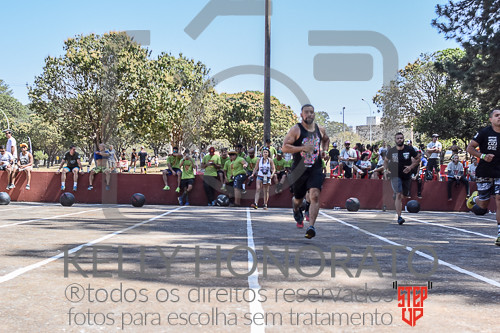The image depicts a casual running event on a track, possibly set in a park area. Three runners, all appearing fit, are in different lanes with one running prominently in the second lane from the right. The atmosphere is laid-back, with numerous spectators casually observing; some are standing while others lean or sit against a mid-length red wall. In the center background, a noticeable group of six to seven people dresses uniformly in green t-shirts. The scene features a few elements like transparent gray lettering across the middle, with "Kelly Honorado" and some Spanish text at the bottom overlaying the image. The backdrop consists of tall, fully bloomed trees, contributing to a vibrant, outdoor setting. Additionally, a "Step Up" logo is visible, adding to the casual yet organized ambiance of the event.